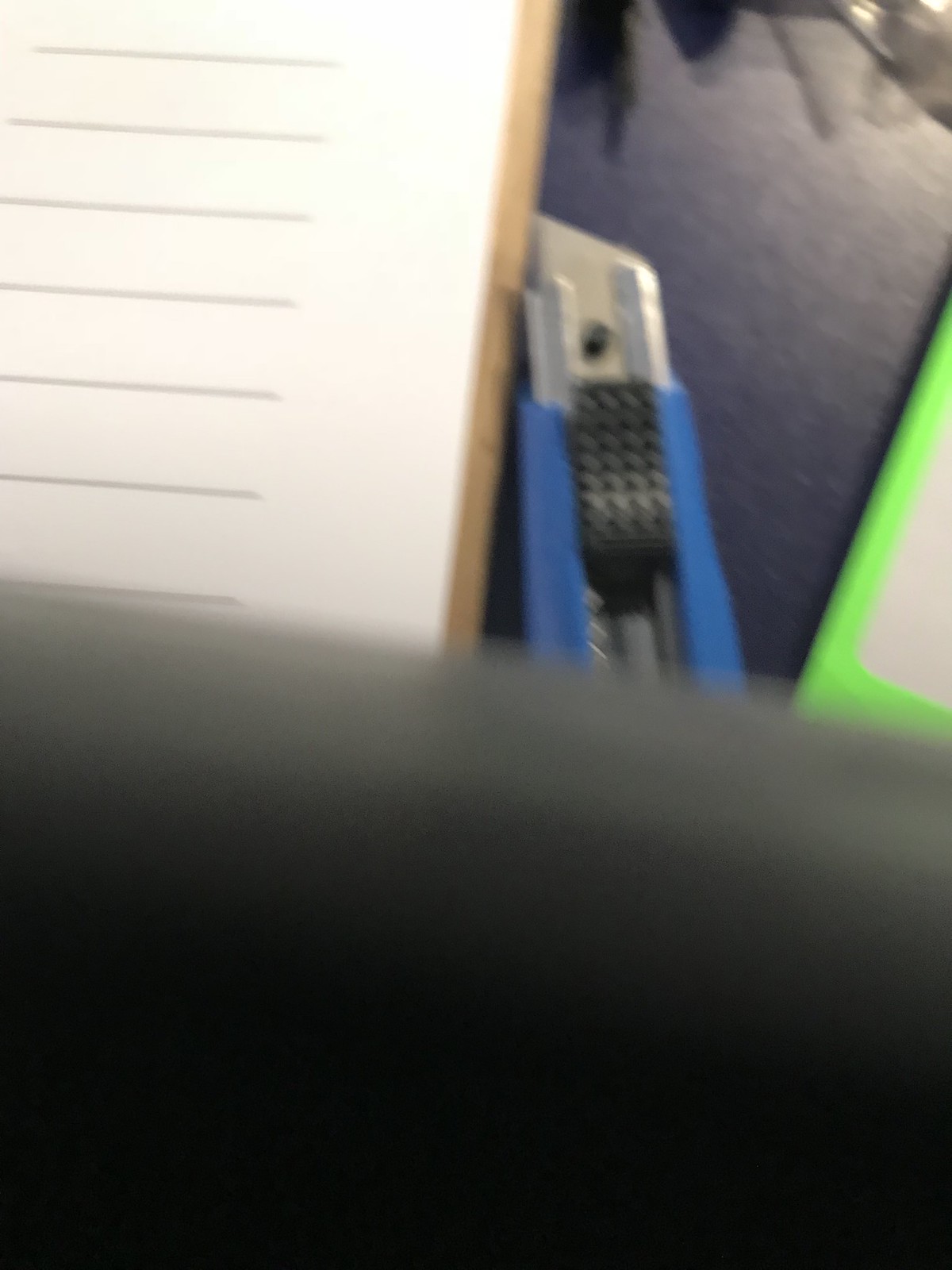This image features an accidental, blurry capture, likely taken with an iPhone or similar smartphone based on its shape and quality. Dominating the center of the photograph is a silver X-Acto knife, identifiable by its unique design with a blue plastic grip and a black plastic knob used to adjust the blade. To the knife's left, there appears to be lined paper attached to a clipboard, indicated by faint hints of tan and white colors. On the right side of the knife, a neon green-outlined object is partially discernible. The backdrop for these items is predominantly black, while the foreground, covering about half of the lower section of the image, shows a solid black area as if something blocked the camera lens.